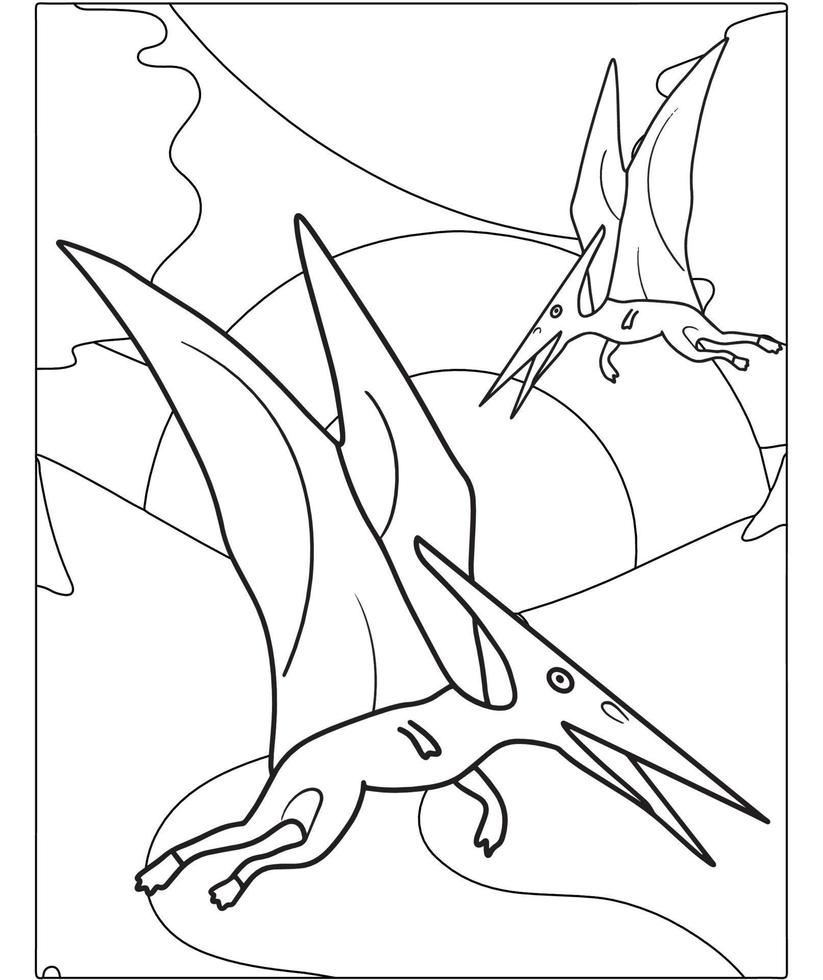The image is a simple black-and-white illustration that resembles a page from a coloring book, drawn with black ink outlines on a white background. It depicts a rather desolate landscape with minimal details. In the background, there is a circular shape likely representing the sun. Below the sun, a few squiggly lines and curved shapes seem to suggest hills and a river meandering through the scene. Dominating the foreground are two stylized pterodactyls flying in the air. 

The pterodactyl in the front is large, its massive, bat-like wings extending high above its body in an upraised position. It faces the viewer directly with an open, slightly curved beak that gives an impression of a smile, adding a touch of humor or mischief to the scene. At the top right corner, the second pterodactyl is seen flying towards the left, its beak also curved in a similar manner. Both pterodactyls are characterized by their long, sharp beaks and elongated heads that taper into horn-like shapes. There are no people or textual elements in the illustration, which focuses solely on the prehistoric creatures and the ambiguous, stark backdrop.